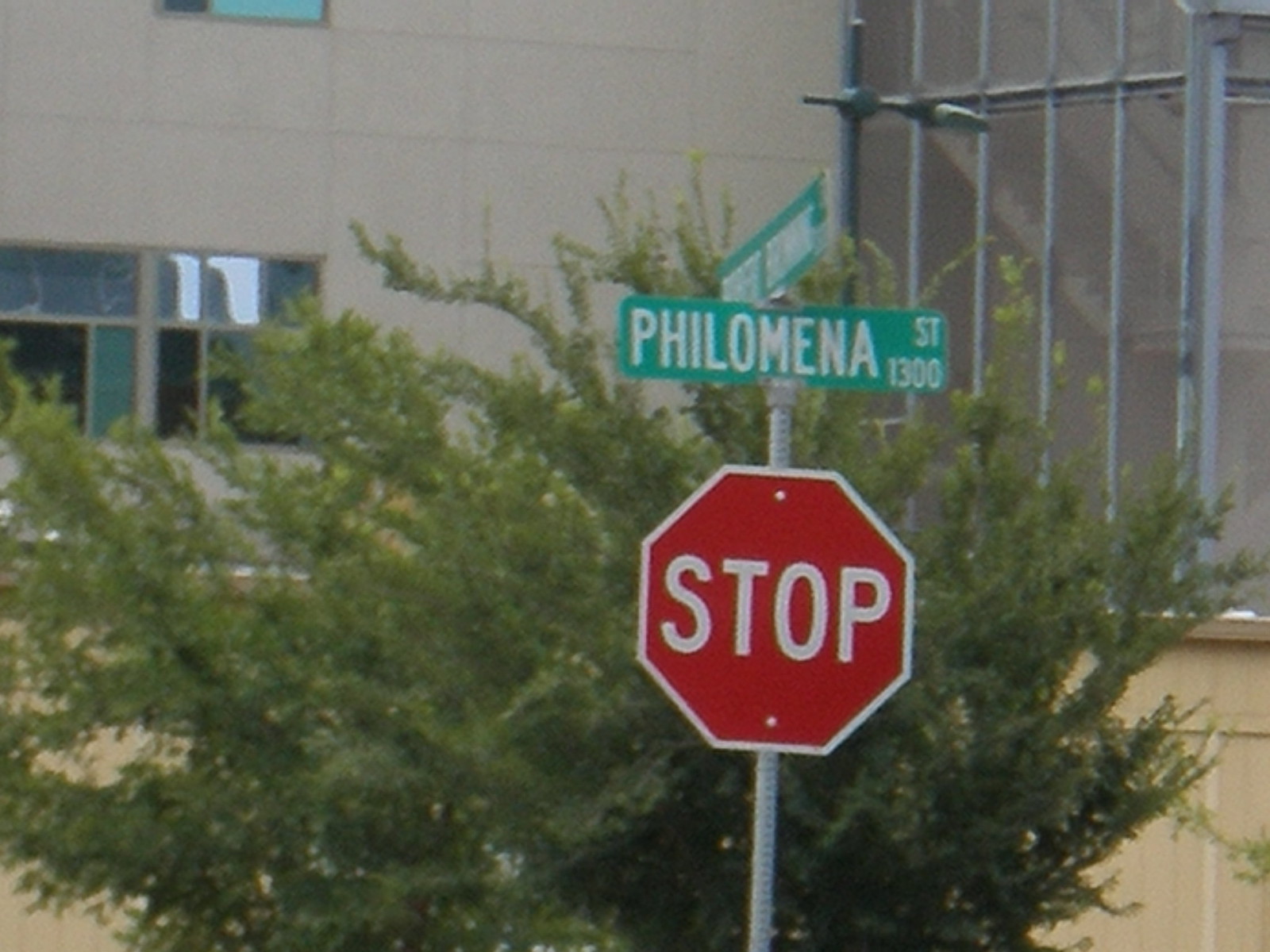In this daytime photograph, the centerpiece is a red octagonal stop sign affixed to a silver metallic pole, located towards the bottom right. The stop sign, bordered in white with the word "STOP" in bold white letters, is attached to the pole with two visible rivets. Above the stop sign, the pole extends upward to display a green street sign with white text reading "Philomena Street 1300." There is an additional street sign at the top, partially turned and unreadable.

Behind the signs stands a large, sprawling, circular-shaped tree with rich green foliage that occupies about three-quarters of the image's height, hinting at a lush background. Further in the distance, there is a building with a light brown facade that transitions to an orangey-brown color towards the bottom. This structure displays a mixture of white wood paneling and windows, some on the very right side and a few open, light blue-barred windows towards the left, indicating an urban setting.